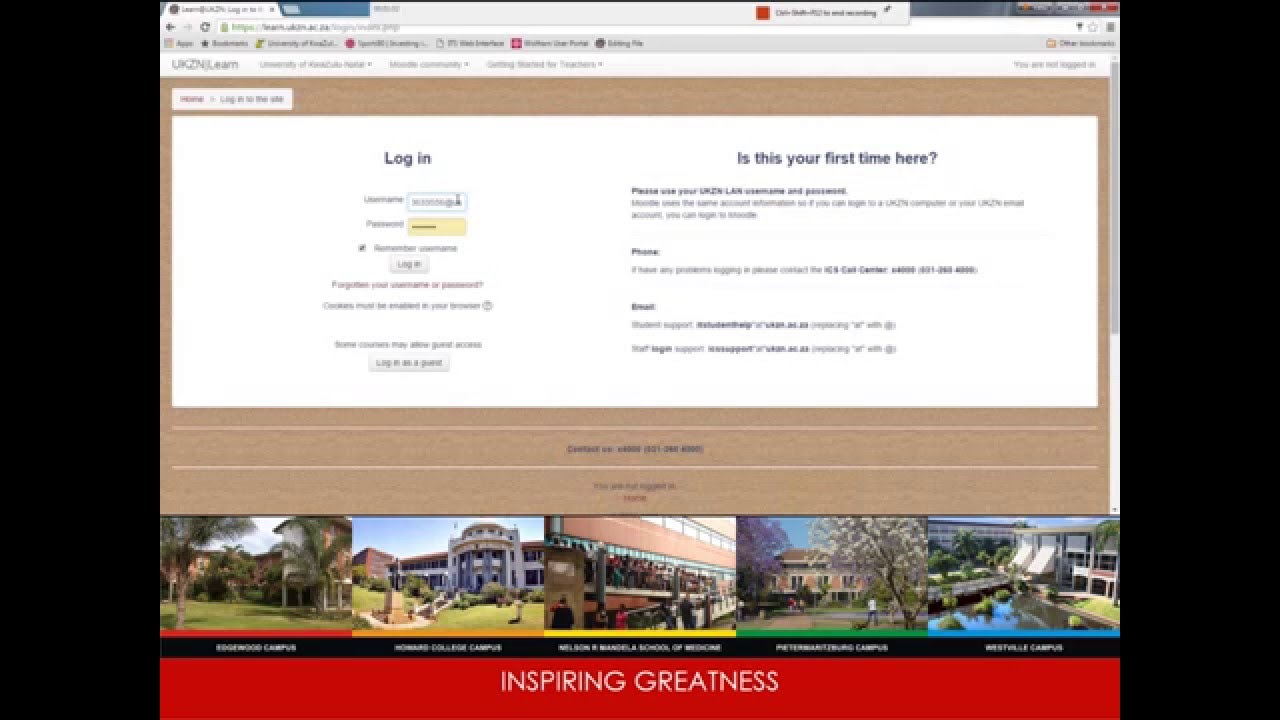**Detailed Descriptive Caption:**

In this image, we're looking at a screenshot likely taken from a Firefox browser, displaying a webpage with multiple layers of content. 

The top of the image features several tabs from the Firefox browser interface, though the specifics of these tabs are somewhat blurred. Directly beneath the tabs, you can see the address bar containing the URL, followed by the browser's menu bar, both of which are also slightly out of focus but still legible.

The main content of the webpage is presented on a white background with a primary navigation area at the top. This section includes the "UNC2Learn" header and various drop-down menu options. Beneath this navigation area is a prominently featured brown box that resembles a wooden texture. 

Inside this brown box, a white section includes the following elements:
- A "Home" link.
- A "Login to the site" option.

The white area of the box is split into two sections:
1. The left section contains the login fields where users can enter their username and password, with an option to remember the username. Additionally, there are login options for "Login" and "Sign in as a guest."
2. The right section addresses new users with the message, "Is this your first time here?" and instructions to use their username and password. It also provides contact options, including phone and email, for further assistance.

At the bottom of this brown box is a blurred section that appears to contain a phone number and additional text that is indistinguishable. 

Following this brown box, the webpage displays a row of five images, each depicting various locations presumably related to a school campus. Descriptions beneath each image provide contextual information:
1. The first image shows a large building with palm trees in front, labeled "Ridgewood Campus."
2. The second image depicts a modern-looking campus with a large building, a well-maintained lawn, and bushes in front.
3. The third image is less clear but appears to show a group of people standing in a long line outside of a building. The caption is too blurred to read.
4. The fourth image features a brick building with trees in front, possibly a dormitory, identified as part of the campus.
5. The fifth image, labeled "Westfield Campus," shows a white building with a lake and a palm tree.

At the very bottom of the image, within a red box, is the inspiring tagline: "Aspiring Greatness."

This detailed description mirrors the structure of the webpage, giving a viewer a comprehensive understanding of the visual and textual elements present in the screenshot.